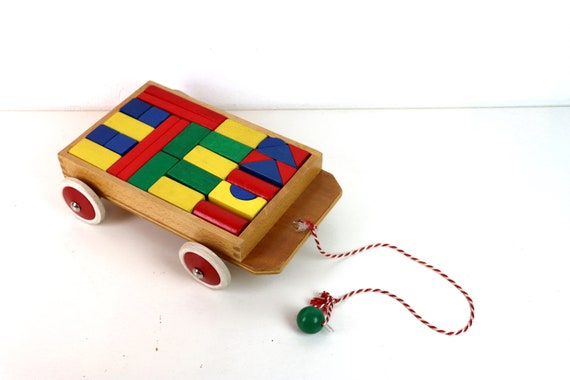This up-close photograph captures a charming, old-fashioned wooden cart toy set against a white surface and background. The cart features two red and white radial wheels with a silver center, and inside the cart, there are various brightly colored wooden blocks. The blocks come in an assortment of shapes, including long red rectangles, blue squares, shorter yellow and green rectangles, blue and red triangles, and a blue half-moon. Each block fits neatly within the cart, suggesting a puzzle-like arrangement for storage. Attached to the front of the cart is a red and white intertwined rope ending in a small green wooden ball, designed for a child to easily pull the wagon along. This detailed and picturesque composition highlights the timeless playfulness and simplicity of a classic child's toy.